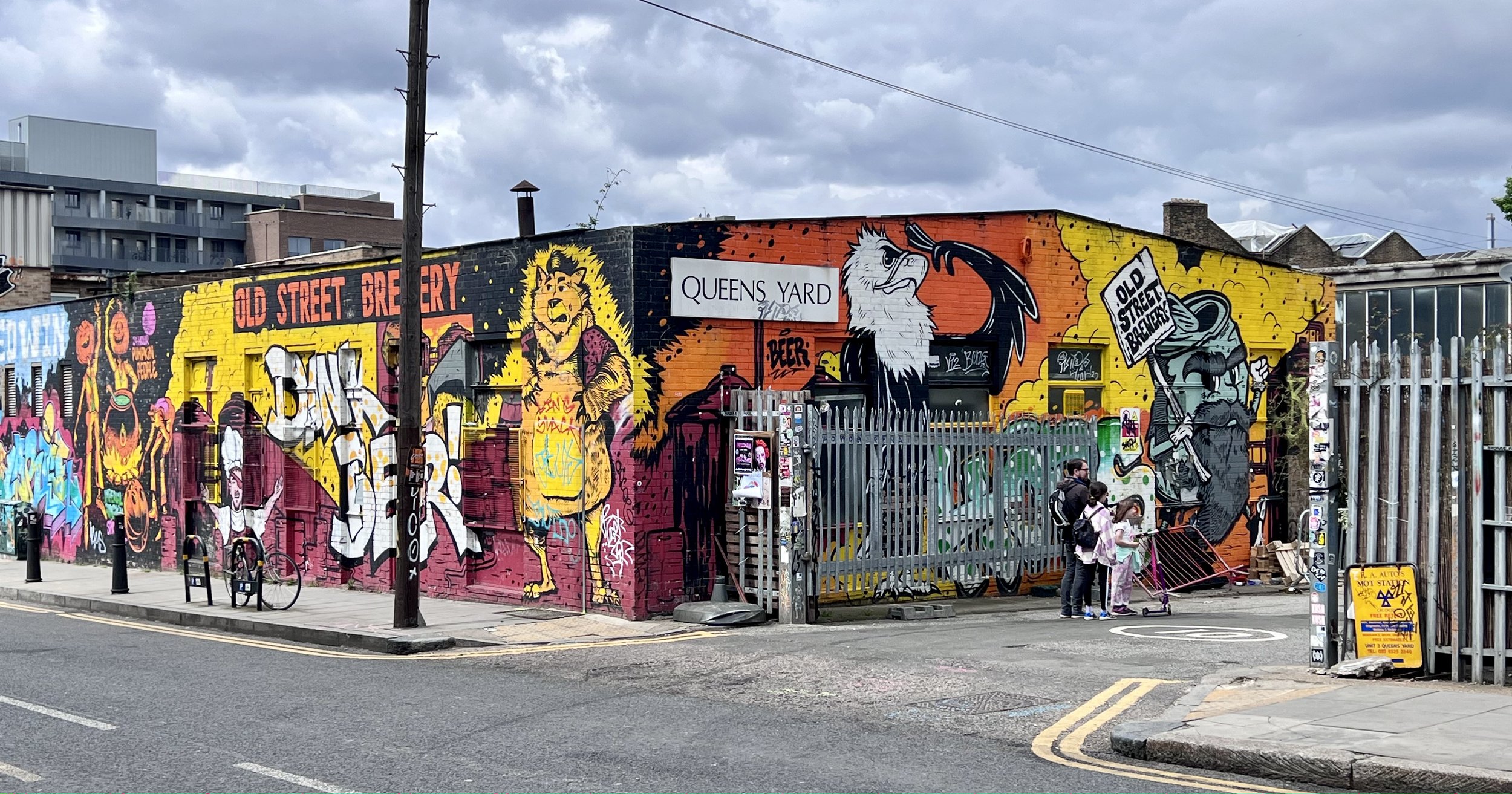The image depicts a vibrant street scene dominated by a unique, one-story business that resembles an A-frame house. This building grabs attention with its expansive mural that adorns the entirety of its exterior walls. The mural is a blend of colorful and detailed artistic elements, featuring a can, a majestic eagle, and a bear standing on its hind legs with a somewhat anthropomorphic appearance. Prominently displayed on a white sign, the name "Queen's Yard" identifies the establishment. To the right-hand side of the image, there is an open gate, with both parts of the gate visible. On the left side of the gate, a section swings open, revealing two individuals standing beside it, adding a dynamic human element to the scene.